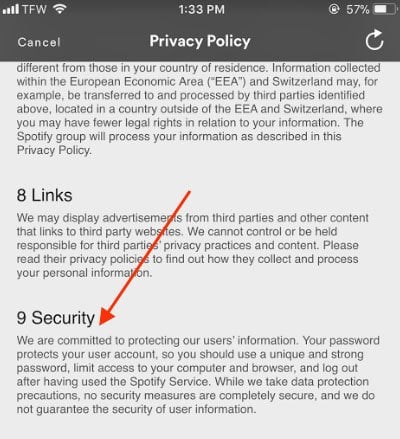This screenshot from a mobile phone displays a section of a privacy policy menu. At the top, a grey banner provides key information: on the top left, full bars of mobile signal accompanied by the text "TFW" in white, and a full WiFi signal; in the center, the time is shown as 1:33 PM; and the top right shows the battery at 57% with a half-filled battery icon. Below the banner, in white font, are the options "Cancel," "Privacy Policy," and a refresh icon.

The main section beneath this header is a grey screen with black text. It starts with the statement "different from those in your country of residence," followed by detailed legal information about data processing in the European Economic Area (EEA) and Switzerland. This text explains how information collected within these regions might be transferred and processed by third parties outside the EEA and Switzerland, where legal protections may be weaker. It assures that the Spotify group will handle the information as outlined in the privacy policy.

Further down, in bold font, the document lists "8. Links," followed by more details, and then "9. Security," which is highlighted by a red arrow pointing at this particular section.